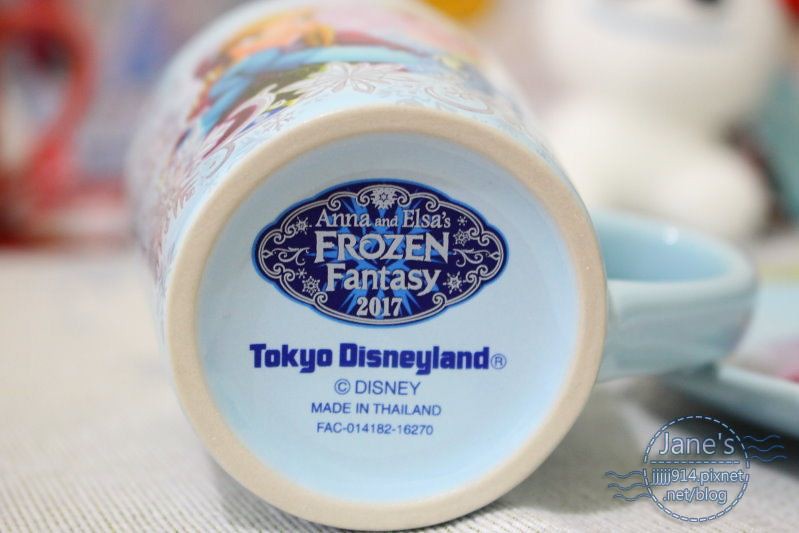This horizontally aligned rectangular image depicts the bottom of a ceramic coffee mug, which is tilted over on its side, with the handle visible on the right side. The mug features a label with elegant, curved, decorative lines and a dark blue circular design, displaying characters Anna and Elsa from the movie Frozen along with the text "Anna and Elsa's Frozen Fantasy 2017" in blue and gold. Below this, additional inscriptions in dark blue include "Tokyo Disneyland," "Disney," "Made in Thailand," and the manufacturing code "FAC-014182-16270." The base of the mug is light blue with a concentric white ring around the edge. The mug rests atop a textured fabric, possibly a placemat. In the lower right corner of the photograph, there’s a logo with the text "Jane's" in the center, underlined by a dashed line, and the URL "914pixnet.net/blog" is also visible.